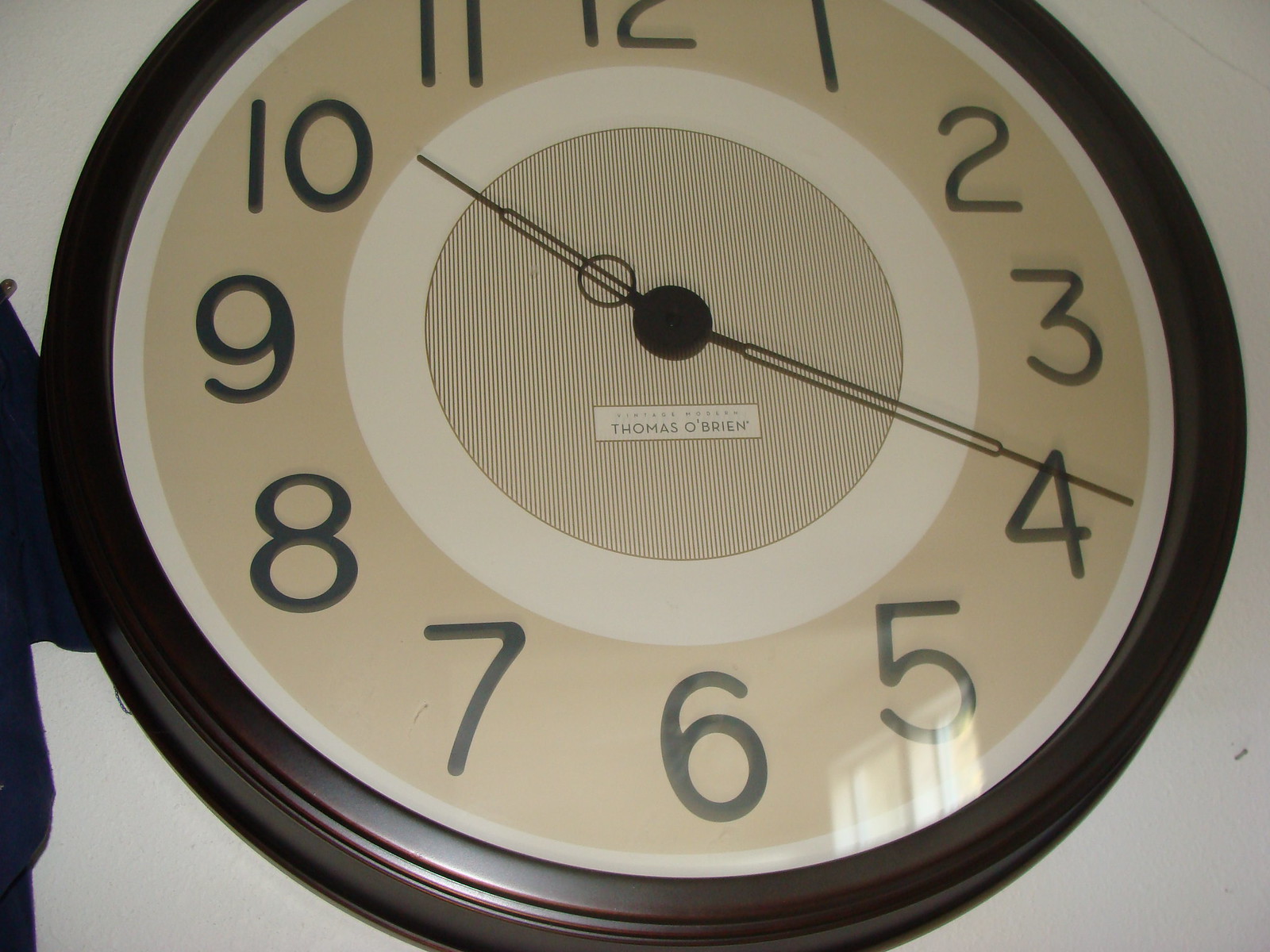The image features a round wall clock with a tan-colored face. The brand name "Thomas O'Brien" is prominently displayed on the clock face. The clock has two black hands: the hour hand is short and pointed at the tip, with a small tube-like section leading to an open circle design; the minute hand is longer and also pointed at the tip, with a thin, elongated tube-like section connecting to the center of the clock. Surrounding the clock face are numbers from 1 to 12, arranged in a traditional circular layout. The clock is encased in a dark brown frame that resembles wood. It is mounted on a light gray wall.